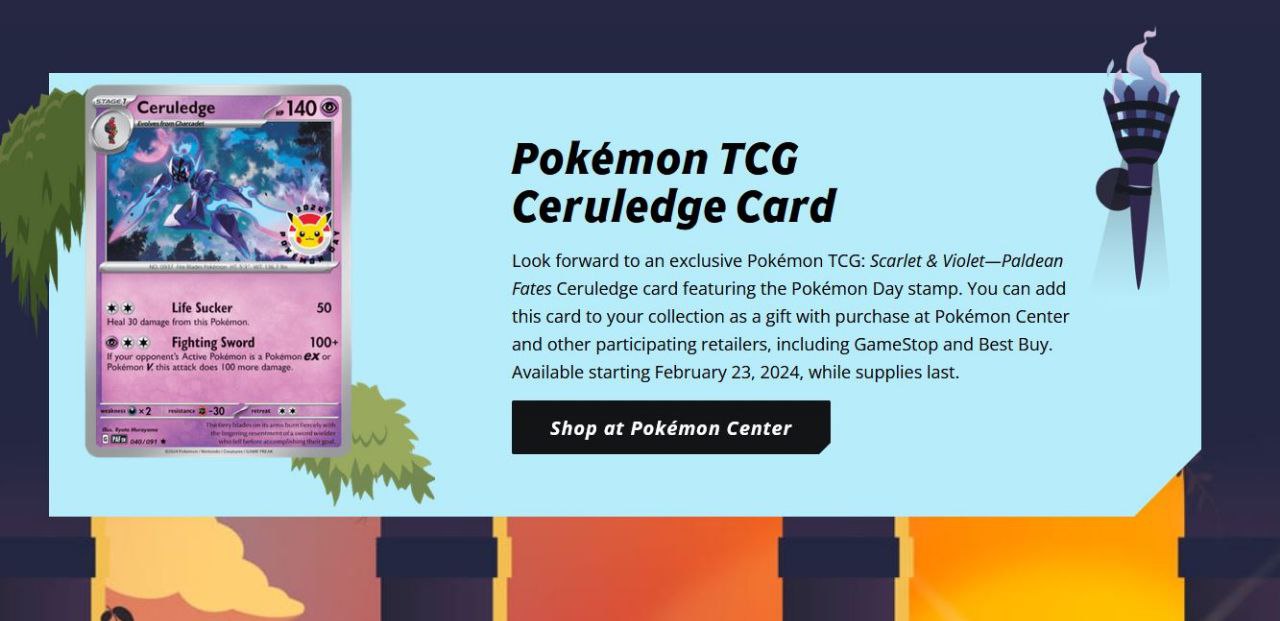In this promotional image related to Pokémon, the overall background is a dark blue. The bottom features three distinct vertical stripes, each with different designs: one filled with clouds, another in a fiery red and orange, and the third in gradient hues of orange and yellow.

Centrally aligned across the image is a horizontal blue rectangle. On the left side of this rectangle, a Pokémon card is prominently displayed. It features "Krillage" with an HP of 140 and showcases an illustration of the Pokémon. The card itself is pink with black text.

To the right of the card, in bold black letters against the blue background, it reads, "TCG Krillage Cards." Beneath this, additional text provides details on the exclusive offering: "Look forward to an exclusive Pokémon TCG Scarlet and Violet Paladin Fates Krillage card featuring the Pokémon Day stamp. You can add this card to your collection as a gift with purchase at Pokémon Center and other participating retailers, including GameStop and Best Buy. Available starting February 23rd, 2024, while supplies last."

Towards the bottom of the image, on a black background with white text, the image prompts viewers to "Shop at Pokémon Center." In the top right corner, there's a blue torch with a striking purple flame, adding a final touch of intrigue to the design.